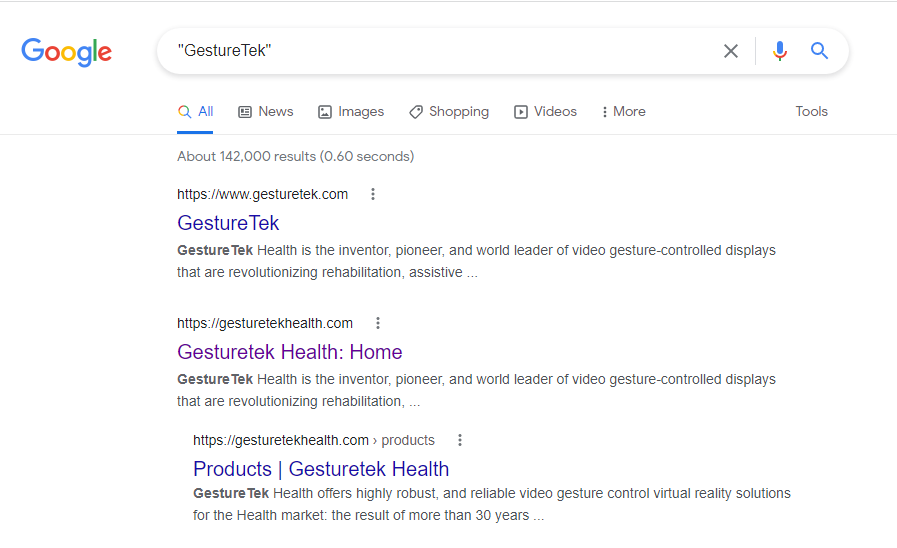The image displays a screenshot of a Google search page on a computer with a white background. In the upper left corner, the recognizable "Google" logo is prominently featured in blue, red, yellow, and green colors. Beside the logo, the search bar contains the text "gesture tech" enclosed in quotation marks. Below the search bar, a navigation menu offers various categories such as "All," "News," "Images," "Shopping," "Videos," and "More," with "All" being highlighted in blue and underlined.

Under this menu, the search results are summarized by a line indicating approximately 142,000 results in 0.60 seconds. The first search result that appears is for the website "gesturetek.com." The entry is headed by the clickable title "GestureTek" in blue text, followed by a description that reads, "GestureTek Health is the inventor, pioneer, and world leader of video gesture-controlled displays that are revolutionizing rehabilitation assistive."

The second search result listed is for "gesturetekhealth.com," with the title "GestureTek Health Home" also in blue text. This description reiterates that "GestureTek Health is the inventor, pioneer, and world leader of video gesture-controlled displays that are revolutionizing rehabilitation." Following this is an indented sub-link labeled "GestureTek Health Products," detailing that "GestureTek Health offers highly robust and reliable video game gesture control virtual reality solutions for the health market, the result of more than 30 years of innovation."